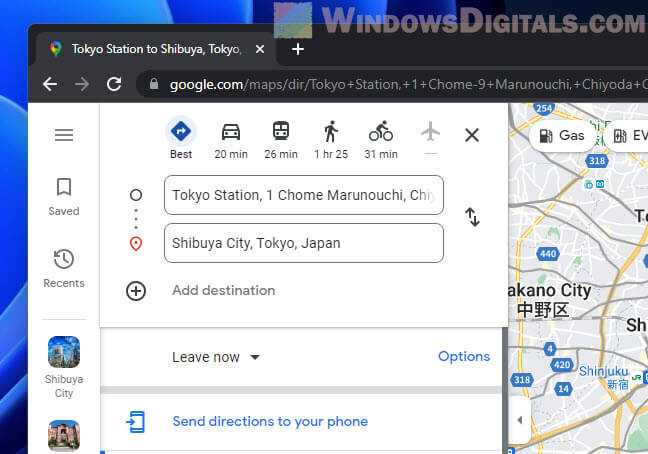Here's a cleaned-up and detailed caption based on your description:

---

This screenshot captures a web page or app interface, specifically, a Google Maps route planning page. In the upper left corner, the browser tab is labeled "Tokyo Station to Shibuya, Tokyo," indicating the current query. It is the only open tab, and a plus sign to its right provides the option to open a new tab. Below the tab bar, navigation buttons are arranged: a back button with a left-pointing arrow, a forward button with a right-pointing arrow (currently grayed out), and a refresh button. 

The URL displayed in the address bar reads: "google.com/maps/dir/Tokyo+Station,+1+Chrome-9+Marunouchi,+Chiyoda". 

On the left side of the screen, a vertical menu comprises three horizontal lines (likely a menu icon), a saved items ribbon, a recent locations clock with a rewind arrow, an entry labeled "Shibuya City," and an image suggesting another city below it.

Dominating the main part of the screen, travel time estimates for various modes of transportation from Tokyo Station to Shibuya are presented: 
- Best route: 20 minutes by car
- 26 minutes by transit
- 1 hour and 25 minutes on foot
- 31 minutes by bike
- Air travel is not an available option for this route.

This detailed interface helps users efficiently determine the best mode of transport for their journey.